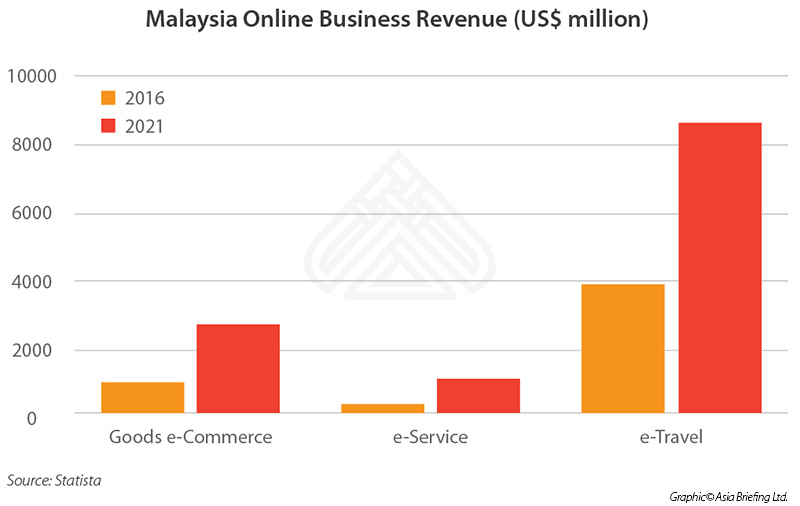This image is a detailed screenshot of a bar graph titled "Malaysia Online Business Revenue (US$ Million)," shown in large, bold black print at the top. The bar graph displays various revenue brackets along the vertical axis, incrementing by 2,000 units from 0 to 10,000. On the right side above the graph, there is a color key indicating two different time periods: orange for the year 2016 and red for the year 2021.

The horizontal axis of the bar graph categorizes revenue sources into three sectors: "Goods and Commerce," "E-Service," and "E-Travel." At the bottom left corner, the source of the data is cited as "Source: Statista," and at the bottom right corner, "Graphic Copyright Asia Briefing Ltd." is noted in very small black print. Intriguingly, a club suit shape is centrally positioned within the screenshot, potentially serving as a decorative or symbolic element.